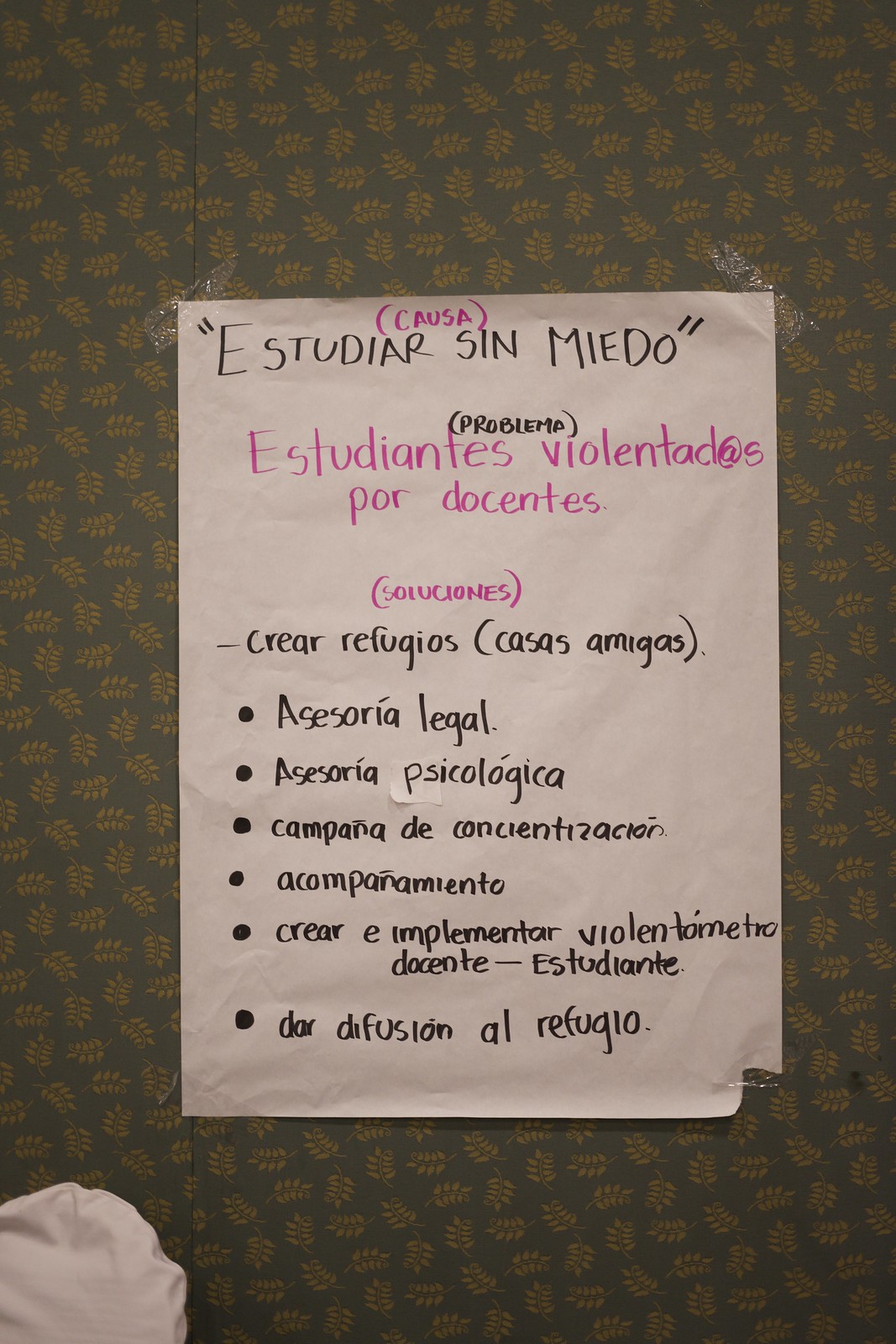The image depicts a piece of paper taped at all four corners to a dark brown wallpaper adorned with gold mini leaves in various directions. The note is written in Spanish with text in black and pink fonts. The title "Estudiar Sin Miedo" (Study Without Fear) is prominently displayed in black. Below this, "Estudiantes Violentades Por Descentes" (Students Assaulted by Descents) is written in pink. The black text continues with "Creer Refugios Casas Amigas" (Believe in Safe Houses), followed by a bulleted list: "Asesoria Legal" (Legal Advice), "Asesoria Psicologica" (Psychological Counseling), "Campaña De Concentración" (Concentration Campaign), "Acompañamiento" (Support), "Creer Implementor Voluntómetro Docente Estudiante" (Believe in Implementing Teacher-Student Volunteering), and "Dar Difusión al Refugio" (Publicize the Shelter). The note also has visibly different formatting and includes handwritten elements, suggesting it was done with a marker. A tear is visible at the lower right corner, revealing part of the floor and a foot, indicating the note may be taped to the floor rather than the wall.